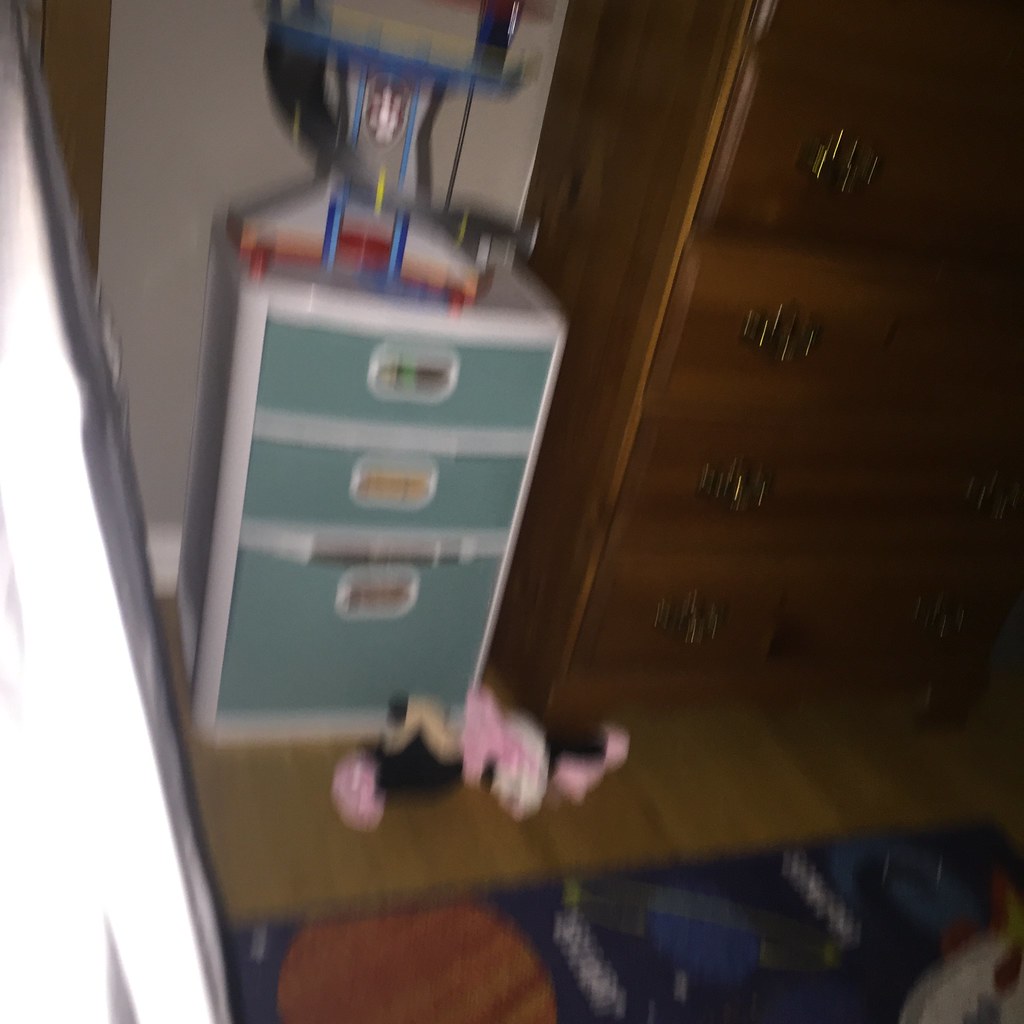In the slightly blurry photograph, the scene is set inside a bedroom. On the left side of the image, there's a small white plastic side table situated next to a bed. This side table features three aquatic blue drawers encased in a white frame, each drawer accessible by sticking your hand into the circular cut-out handles. At the base of the side table, a stuffed Minnie Mouse toy dressed in a pink and white polka dot dress with little pink shoes is prominently displayed. Atop the side table sits a colorful Weebles Wobble toy that includes a circular white track with a blue outline and a red base, encircled by a black plastic track just wide enough for small toy cars to race down.

Adjacent to the side table stands a dark brown dresser, featuring four or five drawers, some of which are slightly ajar, hinting at storage use. Although it's difficult to discern the contents of the side table drawers, various items appear to be stored inside. The overall atmosphere of the room suggests a playful yet organized space, filled with childhood treasures and practical furniture.